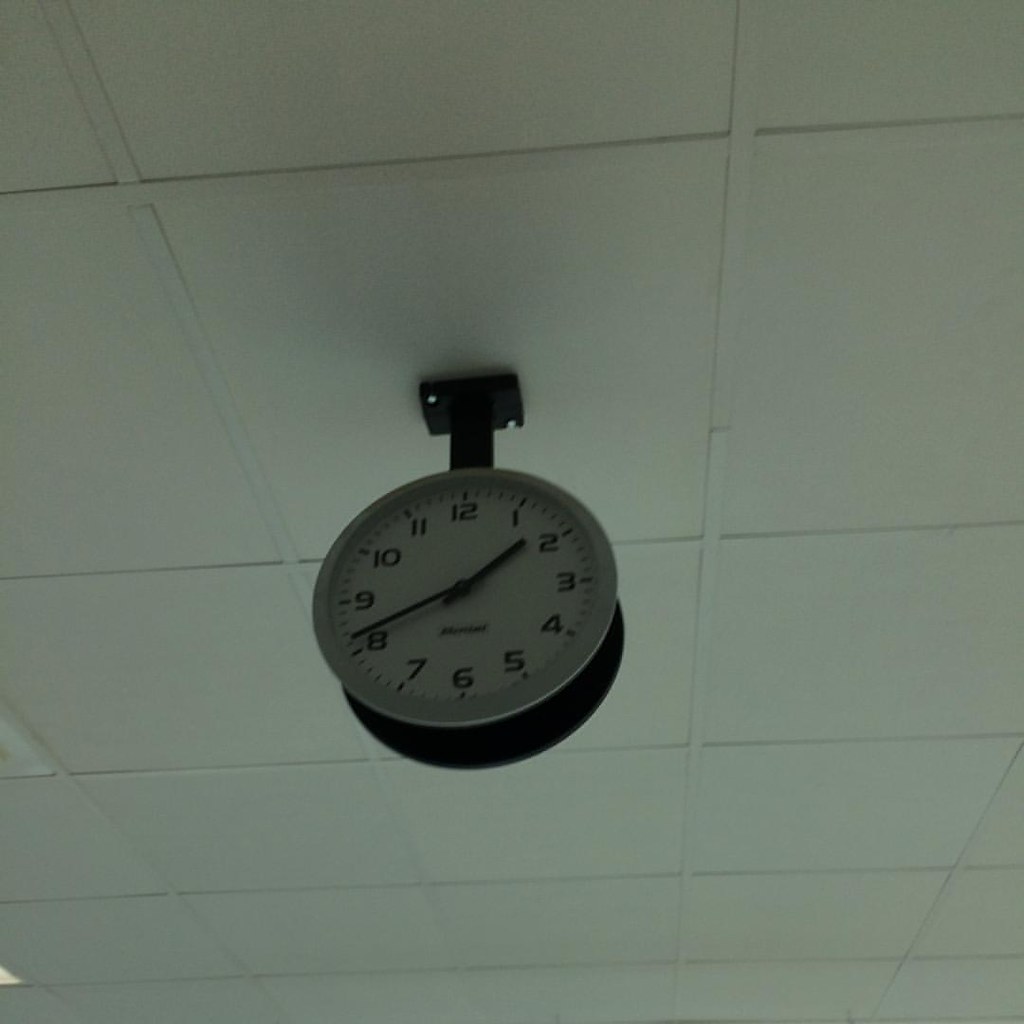This image features a clock suspended from an expansive, white ceiling. The clock is securely attached with two visible silver bolts on either side of its base. The design includes a stem connecting the clock to the ceiling, suggesting the clock is round and robust in its structure. The face of the clock, which is white, might have a counterpart on the other side, indicating a likely two-faced design. Its encasement is bordered with a refined silver edge. Both the hands and the numbers on the clock face are black, ensuring clear readability. The time displayed is approximately 1:41. The ceiling is notably long and devoid of any other elements, emphasizing the clock as the focal point of the image.